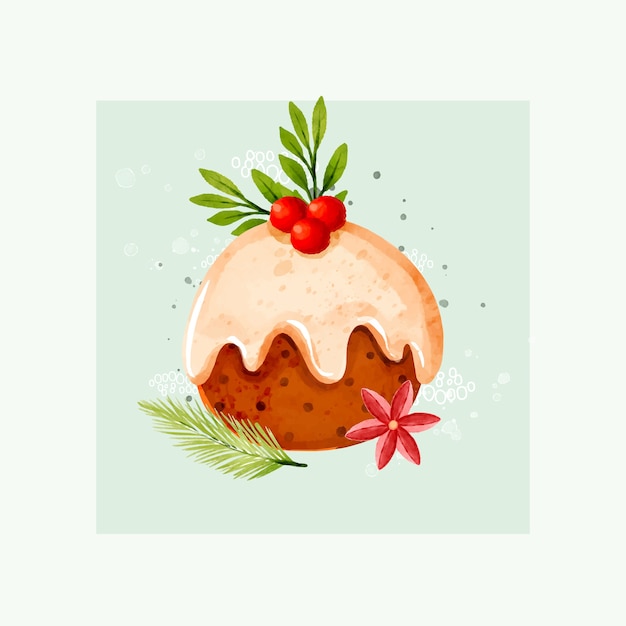The image is a detailed painting of a confectionery item set against a light pastel seafoam green border and a darker green square background. Central to the image is a round, brown dessert adorned with darker dots, and in the foreground is a six-petaled pinkish-red flower situated in the bottom right. The dessert itself appears to be covered in a light salmon-colored frosting or cream that elegantly drips down its sides. On top of this frosting are three red cherries, accompanied by garnishing leaves that add a touch of greenery both in front of and behind the dessert. The lower left corner features a sprig resembling either rosemary or a small pine branch, enhancing the whimsical and delectable appearance of the confection.